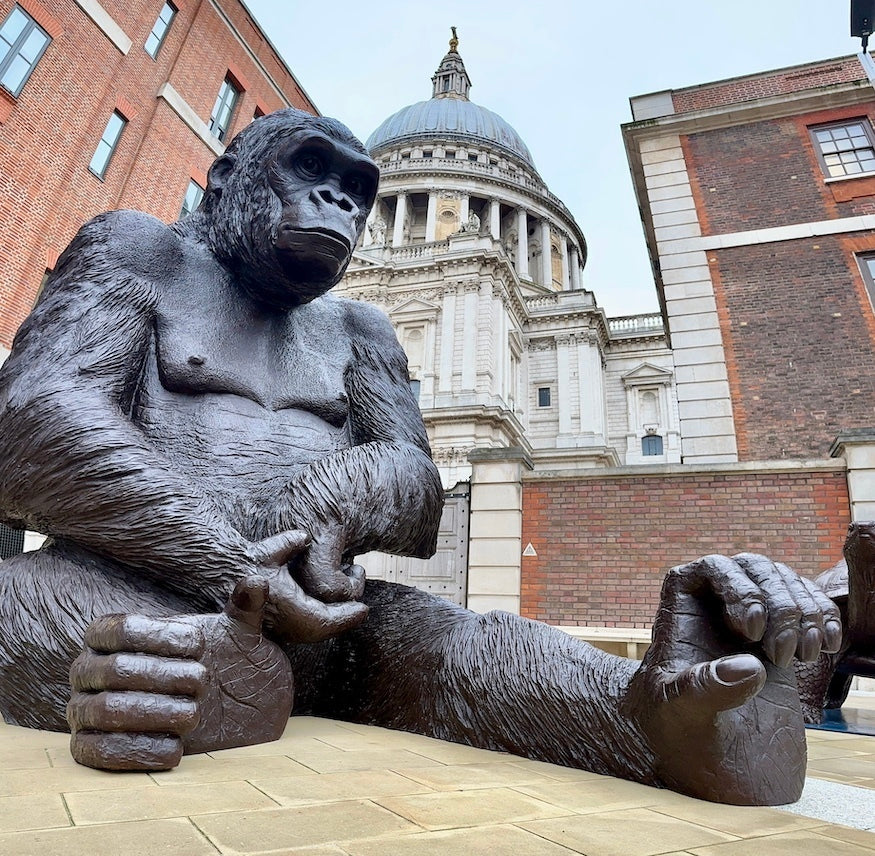The photograph captures an urban courtyard framed by tall buildings: a prominent red brick building, beside which stands a white stone structure with a rounded top, followed by another brick building. In the center of the courtyard sits a detailed statue of a gorilla, seemingly made of stone or metal. The gorilla is posed in a seated position with its feet stretched out in front; the right foot bent inward and the left foot extended with curled toes. The statue's left hand is clenched in a fist, held gently in its open right hand, as the gorilla gazes forward, appearing to look at an unseen observer. Behind the gorilla's right foot, a smaller statue of a turtle or tortoise can also be seen, adding to the artistic assembly in this outdoor space.